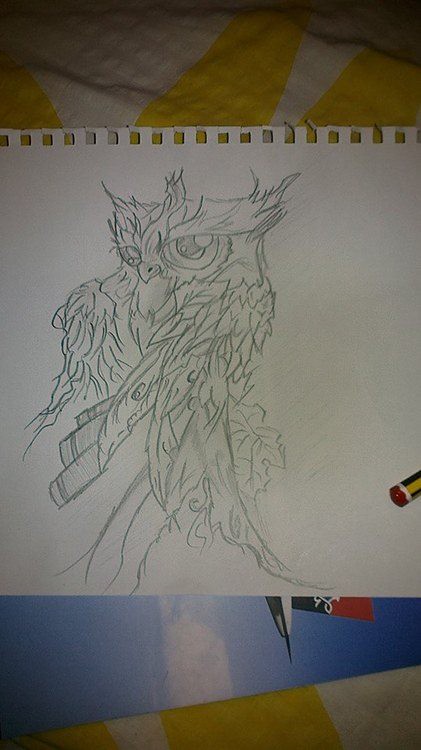The image is a detailed pencil sketch of an owl on a piece of white sketch paper, featuring intricate elements like a wide forehead, large eyes, a small pointed beak, and pointed ears. The owl is depicted with folded wings, sitting on a branch with visible leaves, all rendered in black and white. The edge of the paper appears torn, as if ripped from a notebook. A pen or pencil with a red base, white strip, and black and white body is partially visible on the right side of the paper. Beneath the sketch, there seems to be an overlaid image involving an airplane against a blue sky with white clouds, and beneath that, a table with a mix of white and yellow colors.